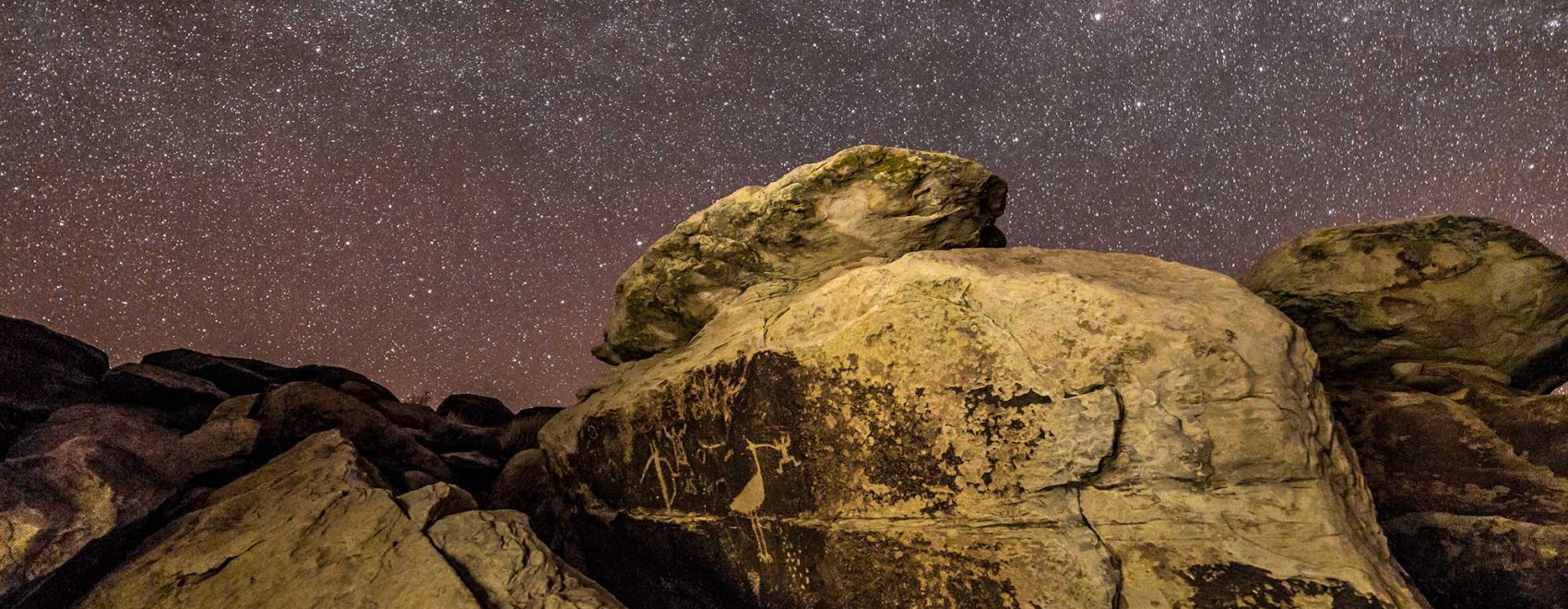The image captures an expansive, thin, wide landscape of a rocky mountain range under a clear night sky. Prominently featuring three large rock formations, the one in the middle stands tallest, flanked by a lower peak on the left and another in the background to the right. The night sky transitions smoothly from a dark purple at the top to a reddish-orange hue at the horizon, filled with a countless array of stars that twinkle brightly. The foreground rocks are illuminated, likely due to a camera flash, revealing their off-gray and yellowish colors. Shadows obscure the details of the rocks in the background. On the leftmost rock formation, faint and primitive cave paintings, though unclear, depict a figure with outstretched arms and legs. The overall scene is serene and majestic, blending the ancient past with the timeless beauty of the night.